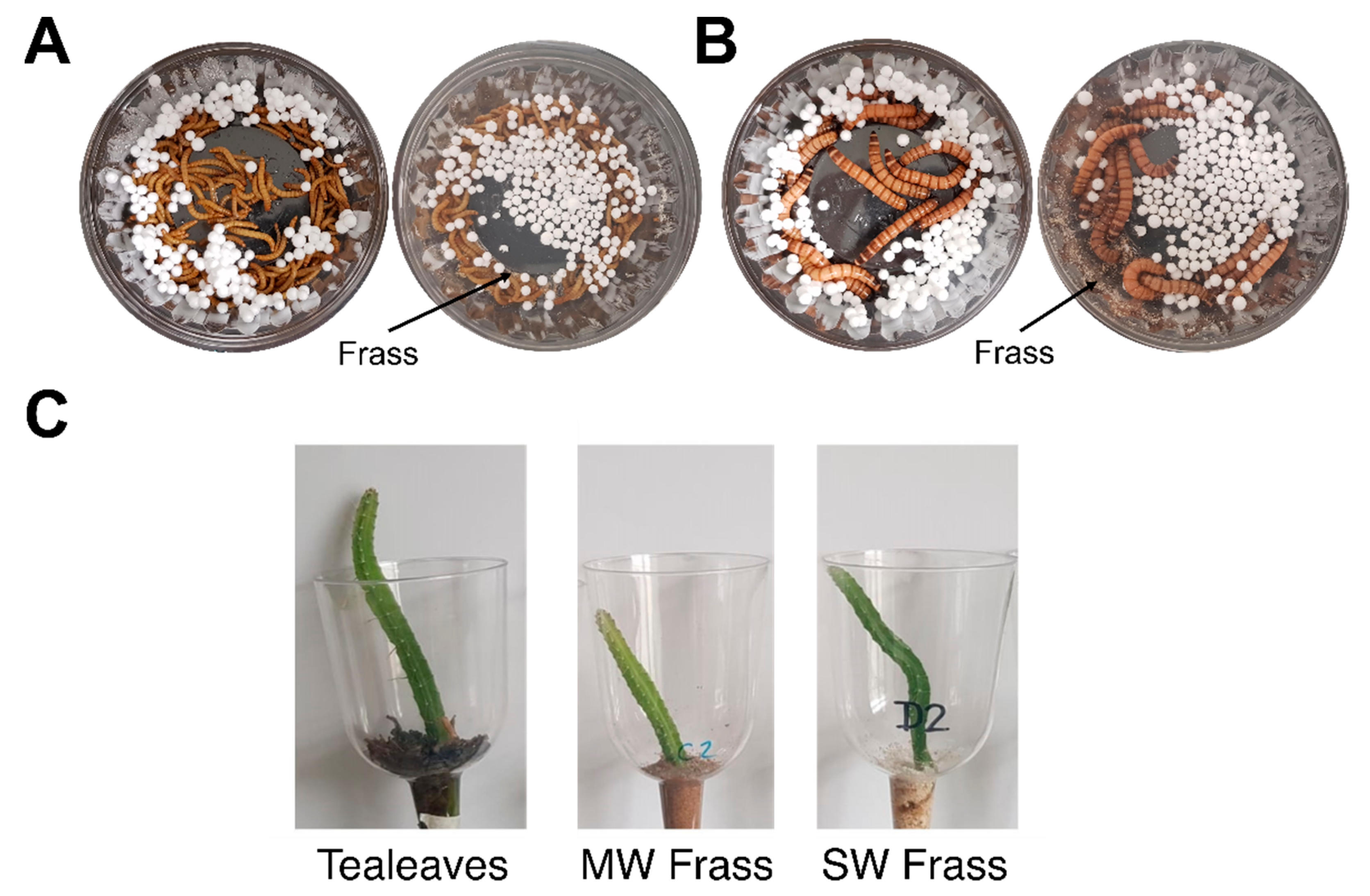The image is a detailed guide on an experimental method for growing cacti using mealworms and frass. At the top, there are four images of petri dishes labeled A and B, showing mealworms and small white granules, identified as frass. The mealworms are used to consume plastic, converting it into frass, a beneficial byproduct for soil. Below these images, there are three glass bulbs labeled C with vibrant cacti growing in them, ranging in color from light to dark green. Each bulb contains different substrate materials: one with cork, one with a brown substance, and one with a black substance. The plant growth is noticeably significant, with descriptions noting that one cactus is long and slightly curled. Each stage of this experimental process emphasizes the transformation from mealworms and frass to successful cactus cultivation in glass containers.